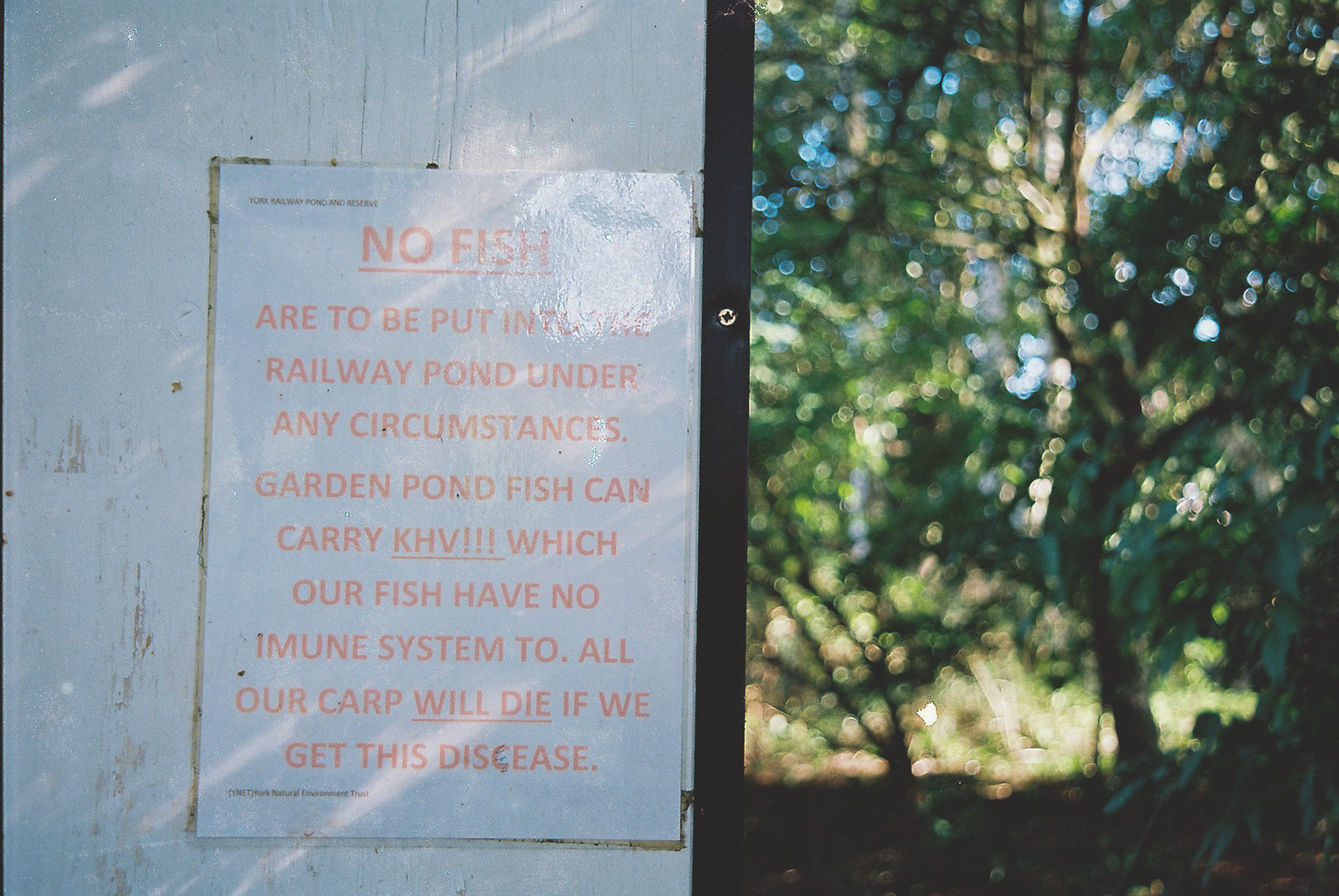The image captures an outdoor scene with a white-painted wooden building on the left side, showing signs of wear with chipped paint and a black border. Affixed to the building's wall, a laminated notice reflects light, indicating its protective plastic covering. The notice, written in large capital letters in a peach or light orange font, sternly declares: "NO FISH" (underlined), followed by "are to be put into the railway pond under any circumstances. Garden pond fish can carry KHV!!!" (underlined), emphasizing the urgency of the message. It further warns, "which our fish have no immune system to. All our carp will die," with the "will die" portion also underlined for emphasis. The right side of the image features a blurry background of dense trees with glimpses of blue sky peeking through the foliage, suggesting the setting is within a forest-like area. The overall atmosphere contrasts the sharp focus on the critical notice against the serene but indistinct natural backdrop.